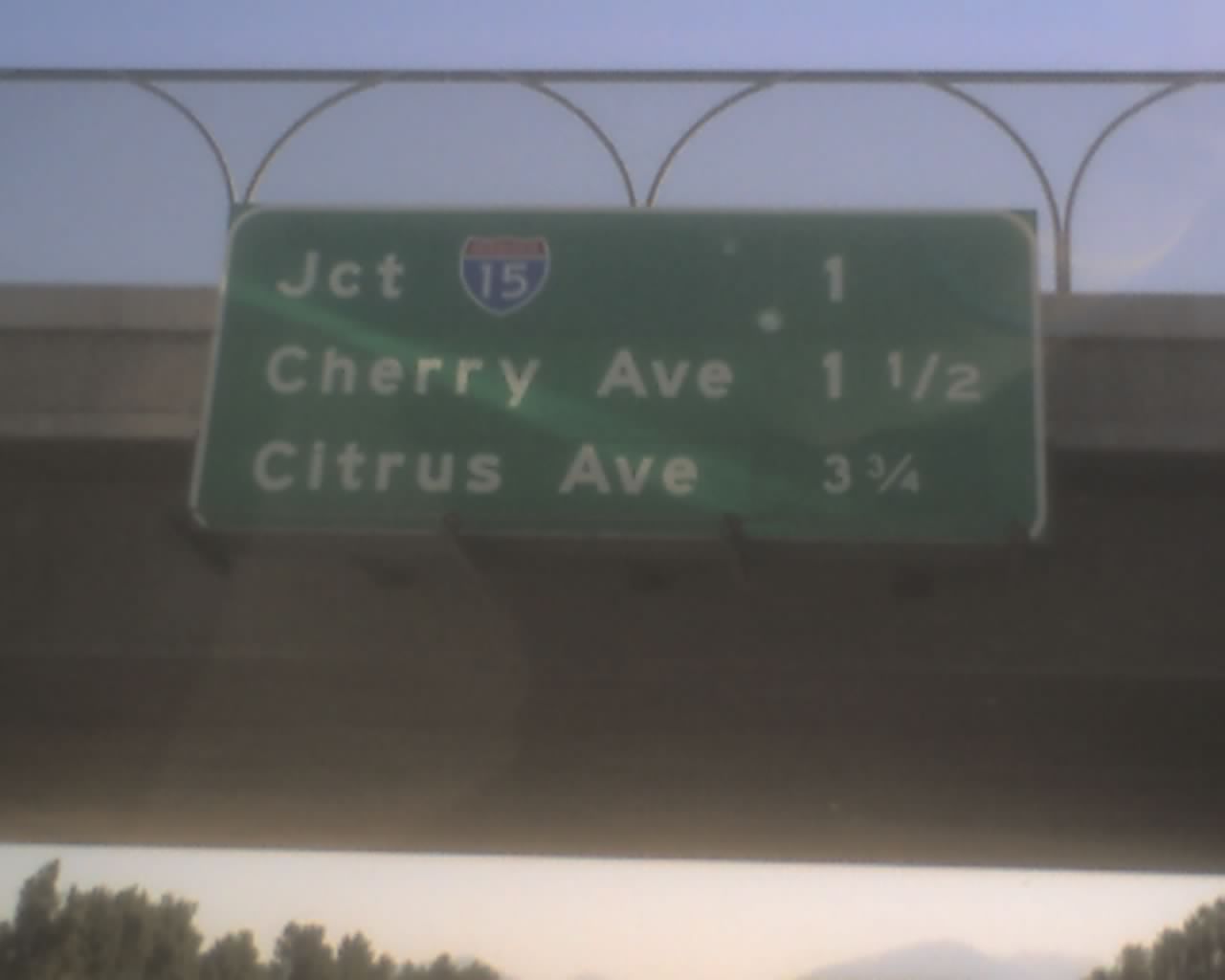This photograph captures a highway sign suspended from a cement overpass, as if viewed from inside a moving car. The sign is a long green rectangle with white lettering, organized into three rows. The top row displays "JCT" alongside an emblem for Interstate 15—a badge-like icon, red on the top and blue on the bottom, with the number 15 in white—followed by the number '1'. The second row reads "Cherry Avenue 1 1⁄2," and the third row states "Citrus Avenue 3 3⁄4." The overpass features a railing with a straight top rail and arched mid-rails. The sky above is blue, suggesting daylight, and the lower part of the image reveals the tops of evergreen trees in both the bottom left and right corners. Additionally, there may be a hint of a hill or mountain range on the horizon, amid a sky that transitions to a yellowish hue near the bottom, possibly indicating sunrise or sunset.